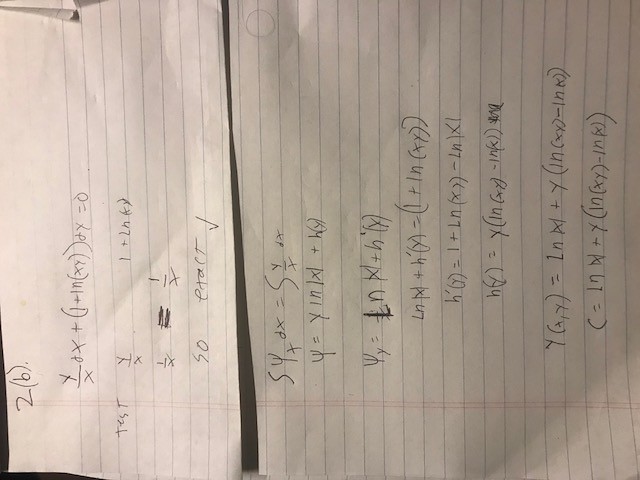This photograph depicts a segment of lined paper with algebraic equations written on it. The paper, featuring a red margin and gray lines, is oriented horizontally and appears to be partially torn, with about the upper quarter separated from the lower three-quarters. The algebraic equations are difficult to decipher due to the sideways orientation, and they seem complex to the untrained eye. The top equation includes variables and expressions such as "x/x," "0x," and "1(1)," arranged in a way that suggests intricate mathematical concepts. Despite the difficulty in interpreting the exact equations, the image clearly captures the essence of a mathematically focused note.